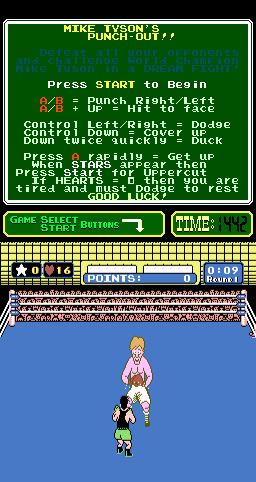This is a detailed screenshot from the classic 1980s video game, “Mike Tyson’s Punch-Out!!”, designed for the original 8-bit Nintendo Entertainment System. The image captures Little Mac in the blue boxing ring, gearing up to face a significantly taller, shirtless, blonde-haired opponent. Little Mac is depicted wearing green shorts and a black tank top. The crowd in the background is colorfully rendered in shades of pink, white, yellow, blue, black, and red.

The top half of the screen features various game controls and instructions against a green background. In bold yellow text, the game title "Mike Tyson’s Punch-Out!!" stands out. It also instructs players that pressing “Start” will begin the game. Specific controls include: A/B buttons for right and left punches, A/B plus up for hitting the face, control left/right for dodging, control down to cover up, down twice quickly to duck, and pressing A rapidly to get up. Additionally, pressing "Start" when stars appear will execute an uppercut. If hearts drop to zero, players must dodge to rest. The screen also displays a timer set at 14:42 and shows two figures in a box, with one noticeably larger than the other.